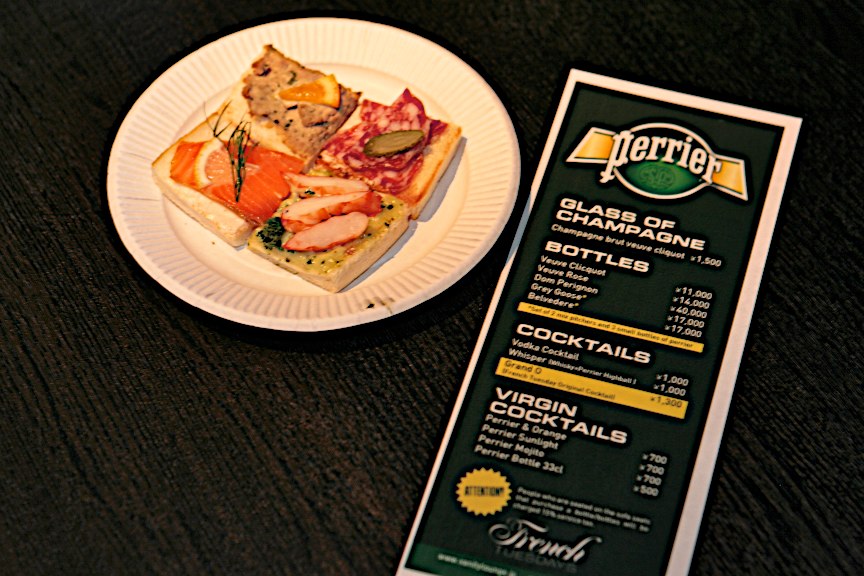The image features a small white plate with delicate lines around the edges, set on a black faux wood table. On the plate are four square pieces of bread, each adorned with different toppings. The first piece, on the far left, seems to have salmon with cream cheese and an orange garnish. The piece at the top left appears to feature some form of brown meat and an orange wedge. The top right piece is topped with salami and a pickle. The piece closest to the viewer is adorned with what seems to be lobster and cheese. To the right of this plate is a long rectangular menu with a white border and a black frame, featuring a dark green interior. The top of the menu prominently displays the Perrier logo, followed by categories including "Glass of Champagne," "Bottles," "Cocktails," and "Virgin Cocktails," each with a comprehensive list of options and their respective prices.